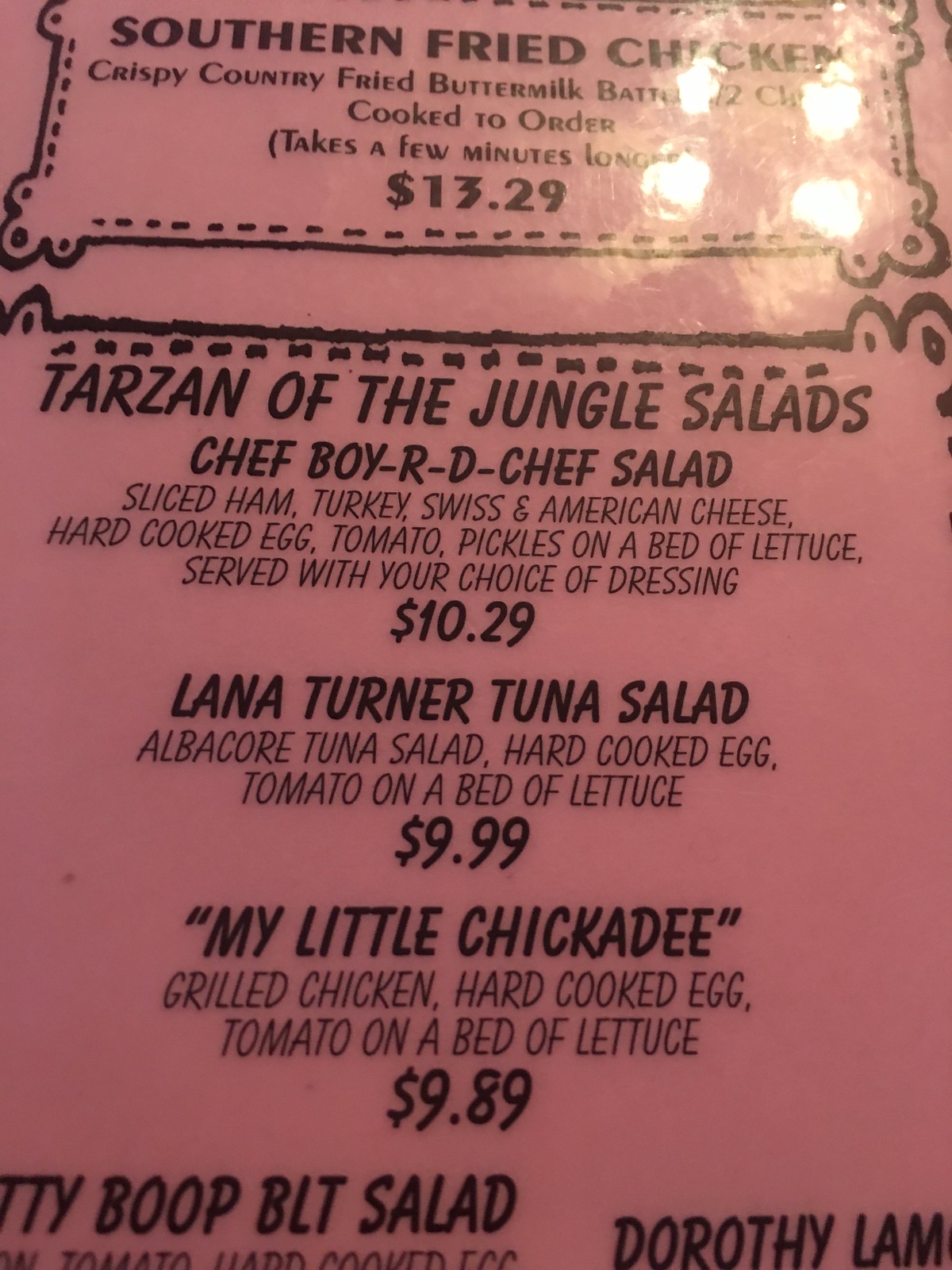This image is a photograph of a vibrant pink menu, featuring decorative border designs and detailed text descriptions of various dishes.

At the top of the menu, approximately an inch from the left edge, a decorative border begins. This border extends downward in a smooth, straight line before curving outward to the left. It then forms a larger curve downwards and to the right, followed by another curve heading rightward. The border straightens again, running close to the edge of the menu. From left to right, the design features a small curve, a larger curve, and finally a smaller curve, extending prominently before terminating beyond the top of the page.

On the right side of the menu, four bright lights create a glare, positioned just inside the edge. The lights are arranged as follows: one is located near the bottom, another directly above that, one to its left, and another below it.

Inside this decorative border, bold black letters read "Southern Fried Chicken." Below this title, in smaller text, it states, "Crispy Chicken Fried Buttermilk Batter," partially obscured by light glare. Further down, it reads, "Cooked to Order" and "It takes a few minutes longer." The price of this dish is listed as "$13.29."

Beneath this section, another border features a similar decorative hump design at its top corners, though the sides extend off the screen. The next segment in large bold letters reads, "Tarzan of the Jungle Salads." Below this heading, individual salad names appear in bold, with descriptions in smaller black text beneath each one. Following the description, each salad's price is highlighted.

In the bottom left corner, entering from the side, large black lettering indicates another dish titled "TTY Boop BLT Salad." Meanwhile, in the bottom right corner, the text reads "Dorothy" with "LAM" trailing off the screen.